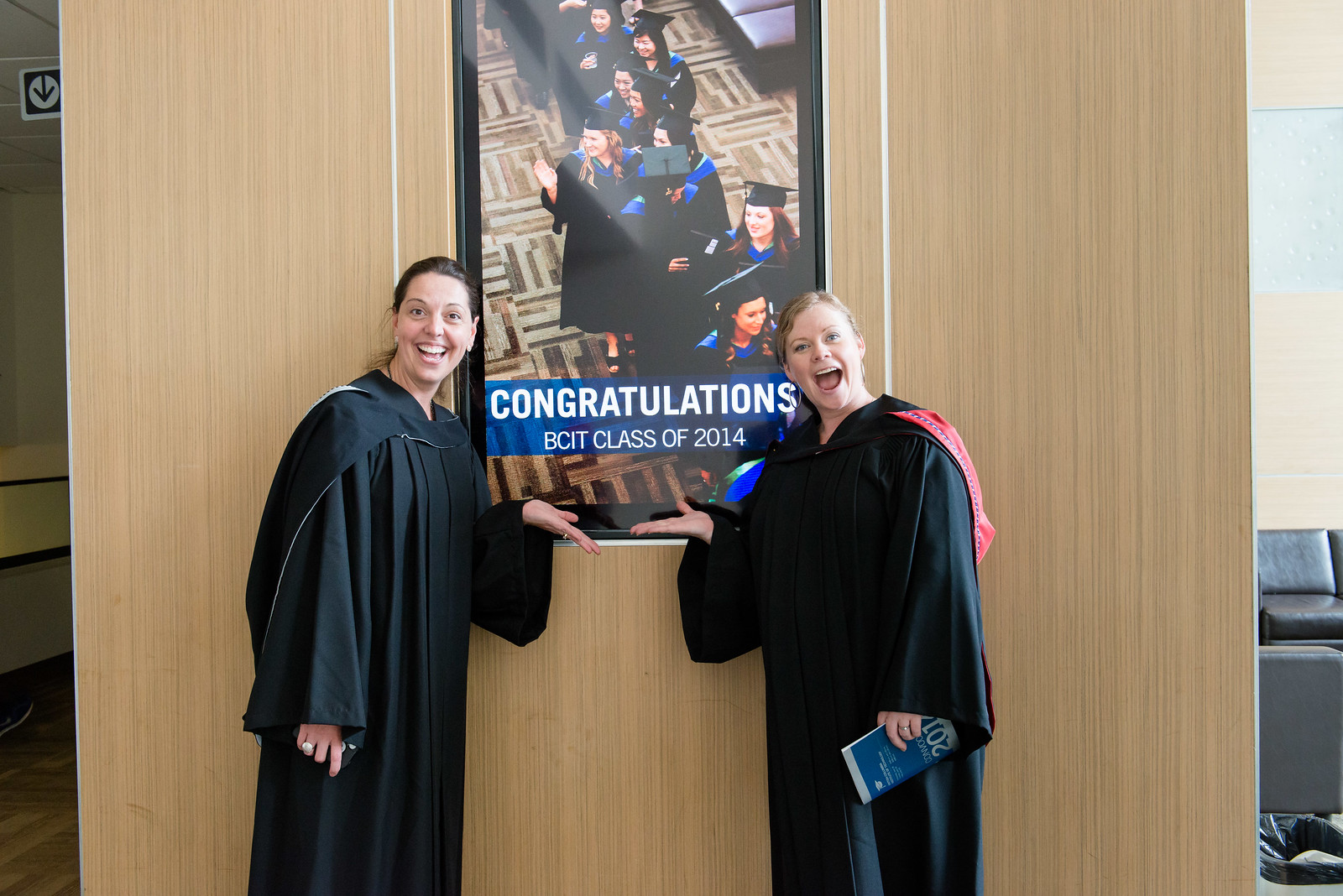This is a detailed photograph of two young women, both wearing black graduation robes, standing indoors in front of a poster that reads, "Congratulations BCIT Class of 2014." The background features beige wood paneling, with an arrow sign in the upper left quadrant and partial seating visible in the bottom right corner. The women are smiling with open mouths, exuding happiness. They both have their hair up and are wearing earrings; the woman on the right has hoop earrings and a wedding ring and is holding a blue and powder blue graduation booklet. The woman on the left also has a wedding ring. They are standing side by side, pointing enthusiastically at the congratulatory poster. The setting includes a hallway and additional seating behind them.